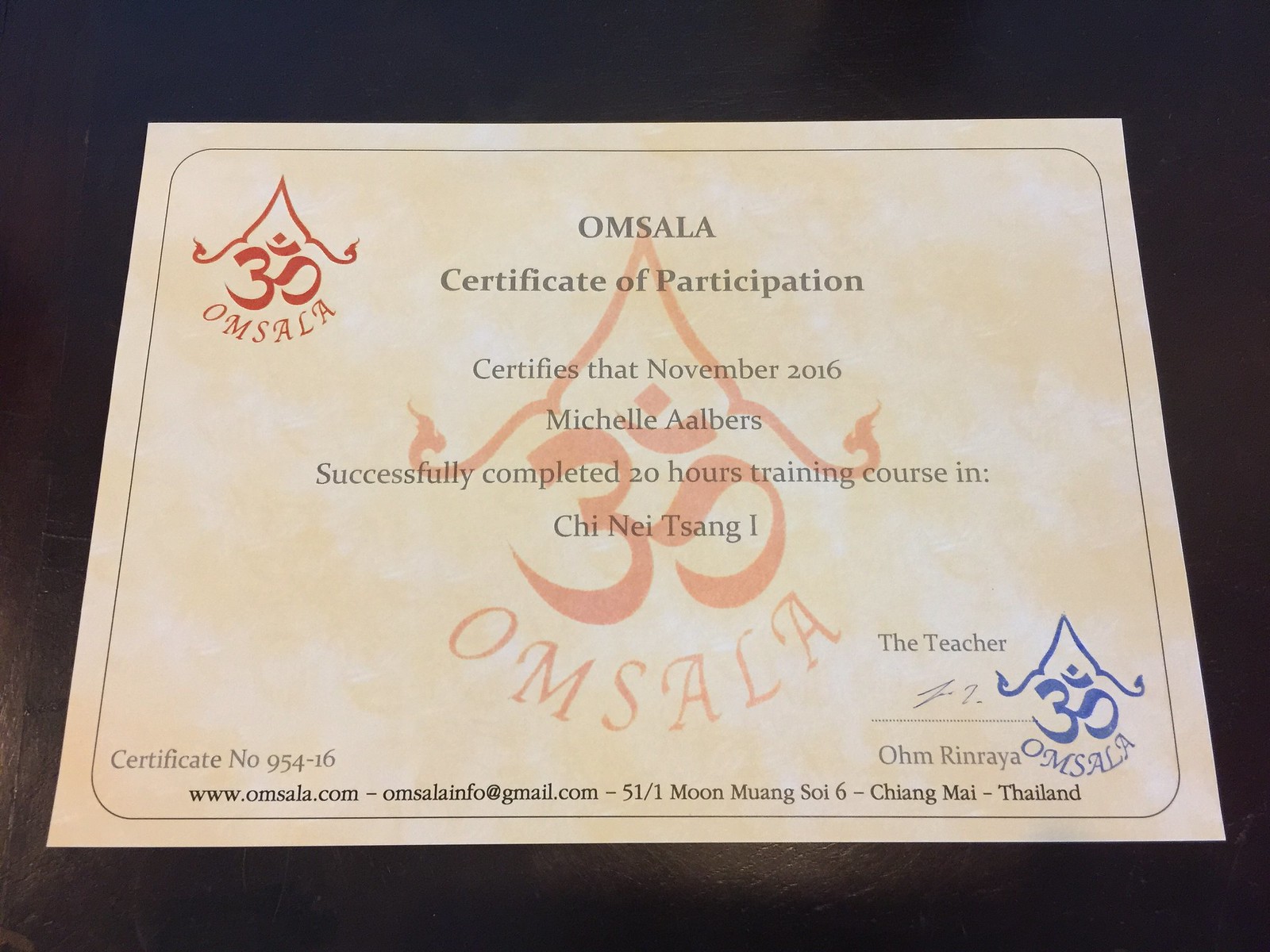The image depicts a Certificate of Participation from OMSALA, set against a black background. The card has a pink hue with a border reminiscent of aged paper in white and yellow tones. In the upper left corner, there is a red logo featuring an Arabic letter resembling a scroll or a "three" with a tent-like shape above it, pointing up. The center of the certificate prominently displays "OMSALA Certificate of Participation" in large, dark print. The text certifies that in November 2016, Michelle Albers successfully completed a 20-hour training course in Chi-Nai-Tsang 1. Below this, there's a large, faint watermark of the OMSALA logo. The lower right corner of the certificate shows the teacher's signature beneath the printed name Rinyana Om, alongside a blue version of the OMSALA logo. On the lower left corner, the Certificate Number 954-16 is listed, and at the bottom, contact information is provided: the website www.omsala.com, the email omsalainfo@gmail.com, and the address 51/1 Moon Muang, Soi 6, Chiang Mai, Thailand.